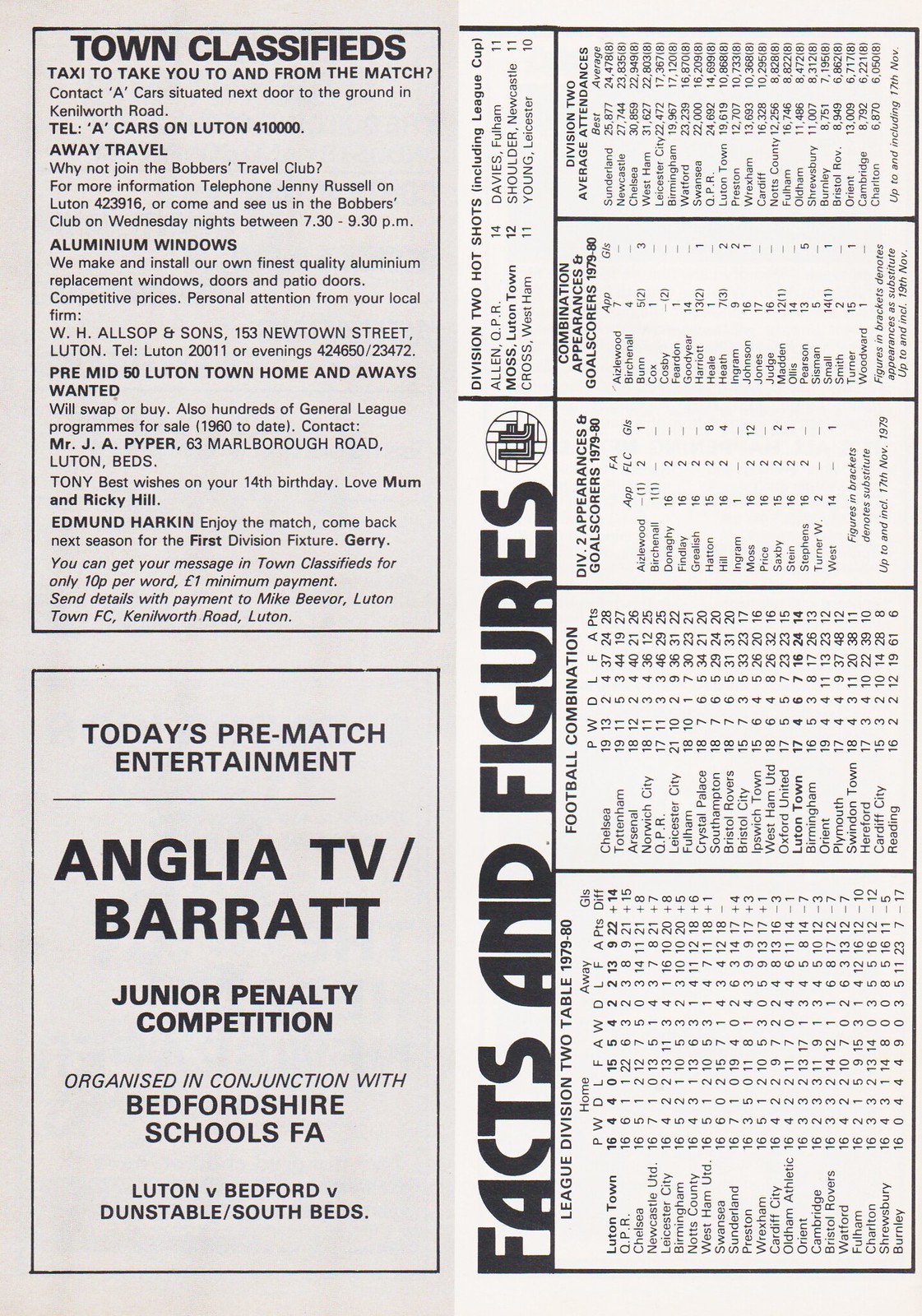The image features a newspaper-like page that combines elements of a sports program and classified ads. On the top left, a section titled "Town Classifieds" advertises services like taxis to take you to and from the match. Below that, it provides details for various local advertisements and lists today's pre-match entertainment. This includes the Anglia TV/Barat Junior Penalty Competition, organized in conjunction with the Bedfordshire Schools FA, featuring teams such as Luton, Bedford, and Dunstable/South Beds. 

The right side of the page is dominated by a vertically oriented chart under the heading "Facts and Figures." This chart includes detailed statistics such as the League Division Two Table for the 1979-1980 season, Division Two appearances and goal scorers, combination appearances, and goal scorers, as well as Division Two average attendance figures. The detailed stats provide insights into different teams' performances in premier league soccer games during that period.